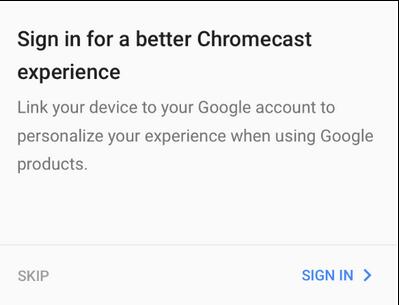The webpage displays a clean, minimalist design with a white background and black text. At the top, there's a bold header in uppercase and lowercase letters stating, "Sign in for a better Chromecast experience." Beneath this header, a smaller, lighter gray text reads, "Link your device to your Google account to personalize your experience when using Google products." A faint line demarcates the end of this instructional text. At the bottom of the page, aligned to the left, is the option to "Skip," while on the bottom right, a blue text button accompanied by a right-pointing arrow invites users to "Sign in." This layout emphasizes ease of navigation and encourages users to link their Chromecast device for enhanced functionality.